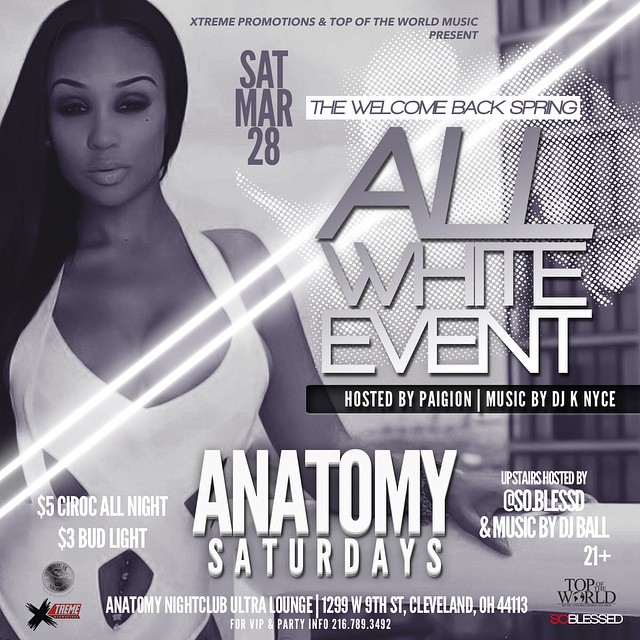This event poster, designed in shades of black, white, and gray, advertises an "All White Event" as part of the Anatomy Saturdays series. The background features a glamorous woman with long dark hair, heavy eye makeup, well-defined eyebrows, and a beauty mark under her left eye, wearing a white, low-cut bathing suit that reveals her jeweled belly button.

Prominent text at the top announces, "Extreme Promotions and Top of the World Music Presents," followed by the event date, "Saturday, March 18th." The event is subtitled "The Welcome Back Spring" and specifies that it is an all-white dress code affair. The event is hosted by PAIGION with music from DJ K Nice, and the upstairs portion of the event is hosted by So Blessed with music by DJ Ball.

Prices for drinks are listed as $5 for CIROC all night and $3 for Bud Light. The venue is "Anatomy Night Club, Ultra Lounge" located at 1299 West 9th Street, Cleveland, OH 44113. The poster indicates the event is 21+ and includes a phone number for VIP and party information: 216-789-3492. Logos for Extreme Promotions and Top of the World So Blessed are located in the corners of the poster.